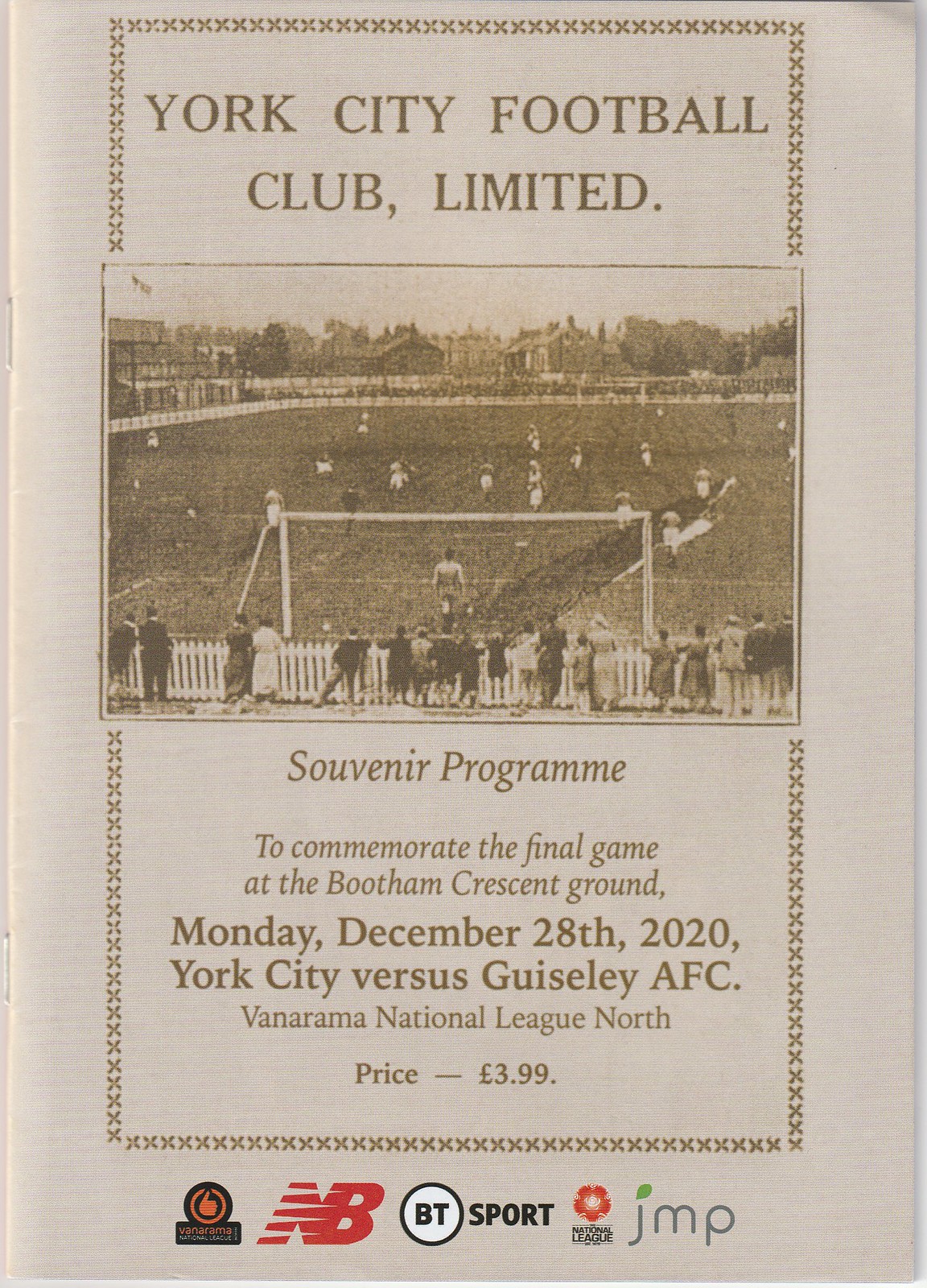The image is a scan or photograph of a program cover printed on lightly yellowed or peach-colored paper. At the top in a bold brown font, it reads "York City Football Club Limited." Centered below this header is a large, black-and-white photograph depicting a football match viewed from behind a football net, which is prominently featured in white. The distant field stretches out with the opposing goal post barely visible. Beneath the photograph, in brown font, is the text "Souvenir Program to commemorate the final game at Bootham Crescent Ground." This is followed by larger letters detailing, "Monday, December 28, 2020. York City vs. Geisley AFC, Vanarama National League North, price £3.99." Surrounding the text and photo is a delicate border made up of small printed X’s. At the very bottom of the cover are several logos in color, including a red New Balance logo and others in multiple colors, serving as advertisements.